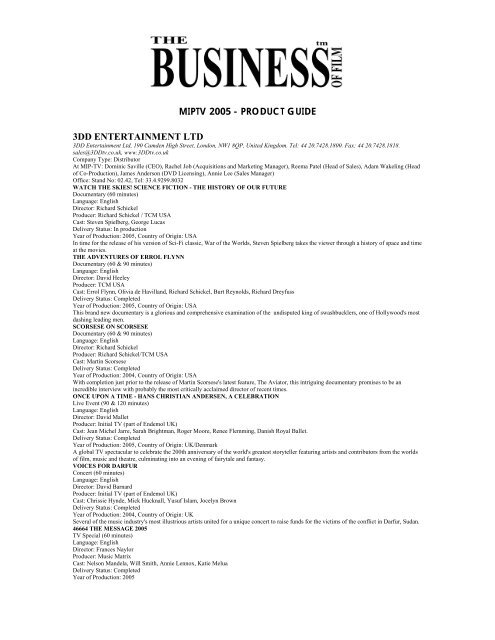The image depicts a page from an industry publication, possibly a magazine or a product guide, featuring a white background with black text. At the very top, it prominently displays "The Business of Film" with "the" in a smaller font at the top left of "Business," which is in a large, bold font. Beside it, "of Film" is written vertically along the last "S" in "Business," from bottom to top. Above "of Film" is the trademark symbol "TM." Below this, the text reads "MIPTV 2005 Product Guide" in black.

The page lists various categories and sections, starting with "3DD Entertainment Ltd." followed by several subheadings such as "Watch the Skies," "Science Fiction," "The History of Our Future," "The Adventures of Errol Flynn," "Scorsese on Scorsese," "Once Upon a Time," "Hans Christian Andersen: A Celebration," "Voices for Darfur," and "The Message." Each section details TV specials, including information about the documentary, director, producer, language, cast, year of production, delivery status, and other relevant details. Some areas are bolded, but due to the small text size, these details are not easily readable.